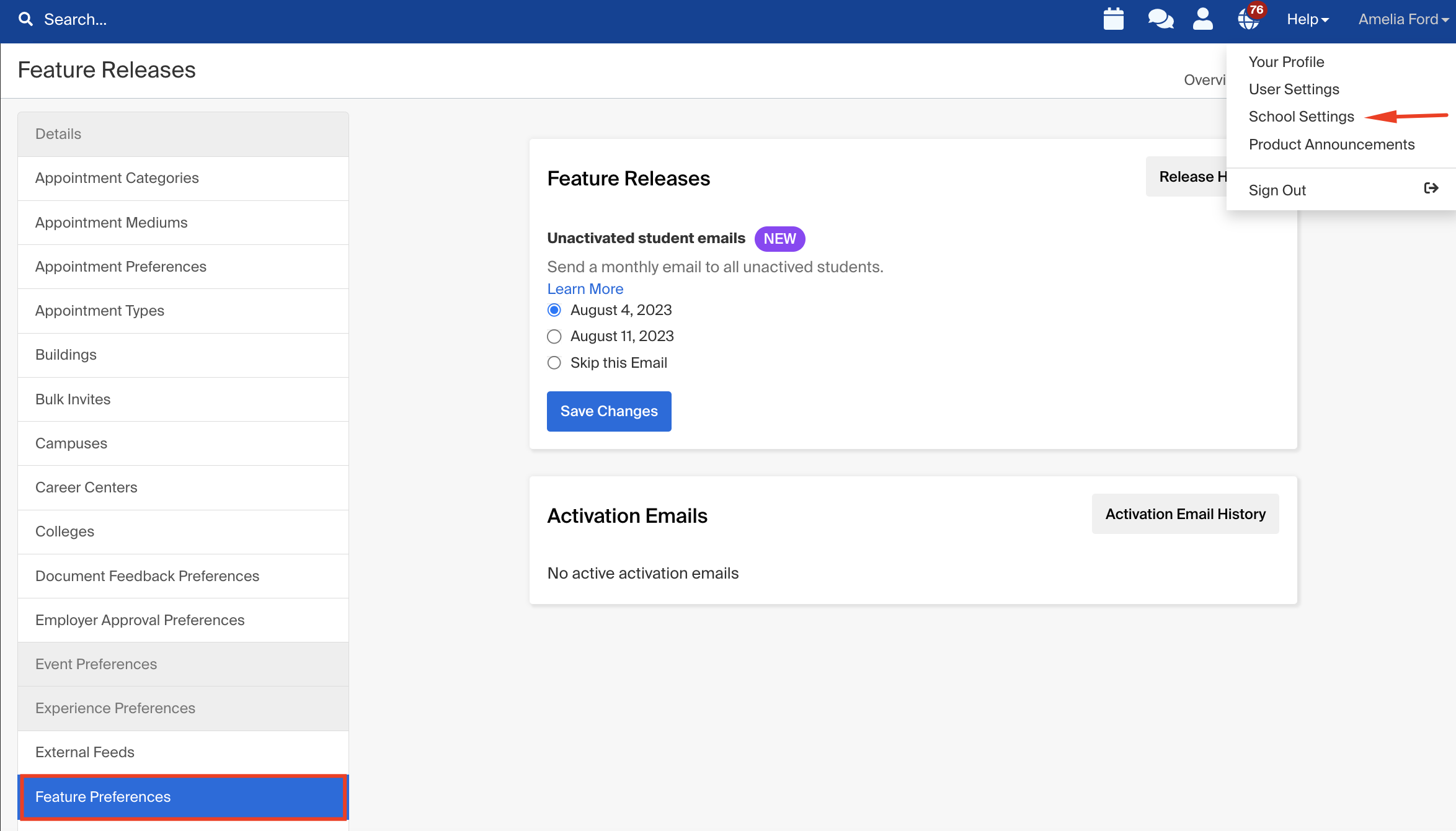Screenshot Description: Interface of an Academic Management Portal

The screenshot depicts a detailed interface of an academic management portal. At the top of the page, there is a blue navigation bar. On the left side of this bar, there is a "Search" label, accompanied by various icons, including a notepad, chat bubbles, a profile icon, and an earth-shaped notification icon with the number "76" displayed in red. Adjacent to these icons, there is a "Help" link, which when clicked, reveals further options: "Your Profile," "User Settings," "School Settings" (highlighted with a red arrow), "Product Announcements," and "Sign Out." 

Beneath this blue bar, the left-hand side features a sidebar titled "Feature Releases," listing multiple categories in blue text within a red outlined box. These categories include: "Details," "Appointment Categories," "Appointment Mediums," "Appointment Preferences," "Appointment Types," "Buildings," "Bulk Invites," "Campuses," "Career Centers," "Colleges," "Document Feedback Preferences," "Employee Approval Preferences," "Event Preferences," "Experience Preferences," "External Feeds," and "Feature Preferences."

In the central portion of the page, the header "Future Releases" is prominently displayed in black. Below this header, an item termed "Unactivated Student Emails" is visible alongside a purple "New" button. The description below briefly mentions sending monthly emails to all unactivated students and includes a "Learn More" link in blue. There are two dates, August 4th, 2023, and August 11th, 2023, each with corresponding buttons. The August 4th date has a checkbox selected, and there is an option to "Skip This Email."

Further down, a blue "Save Changes" button is prominently positioned. There is also a section labeled "Activation Emails" with a button for "Activation Email History" on the right side. Underneath "Activation Emails," it is noted in lighter font that there are no active activation emails. Nearby, another button next to "Future Releases" suggests there is a release function available.

The overall interface appears comprehensive, aimed at managing various aspects of an academic institution's operations with detailed options and settings for user customization.